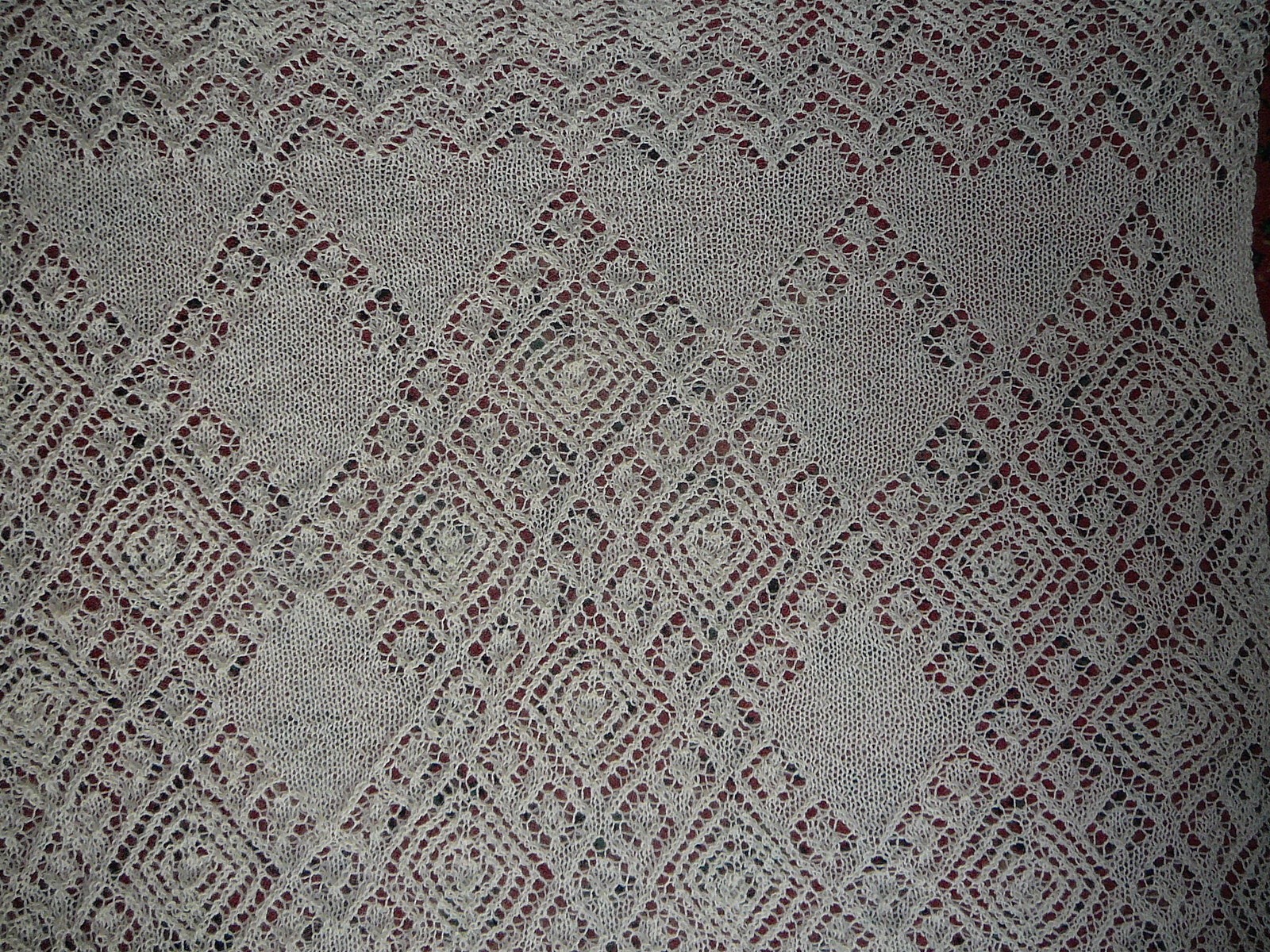This image features a delicate, intricate white doily, likely handmade, displayed prominently. The doily is spread out on a wooden table, with the wood's texture visible through the ornate openings in the fabric. This exquisitely crafted piece consists of a variety of patterns, including diamond shapes, wave-like designs reminiscent of the ocean, and numerous intricate sections with squares within squares and interconnected triangles. The fabric, possibly old, shows slight stretch marks, indicative of its age and handmade nature. The entire image is dominated by this elaborate doily, with its detailed stitching and lacy texture standing out against the background. The setting suggests an indoor environment, with nothing else present on or around the doily.